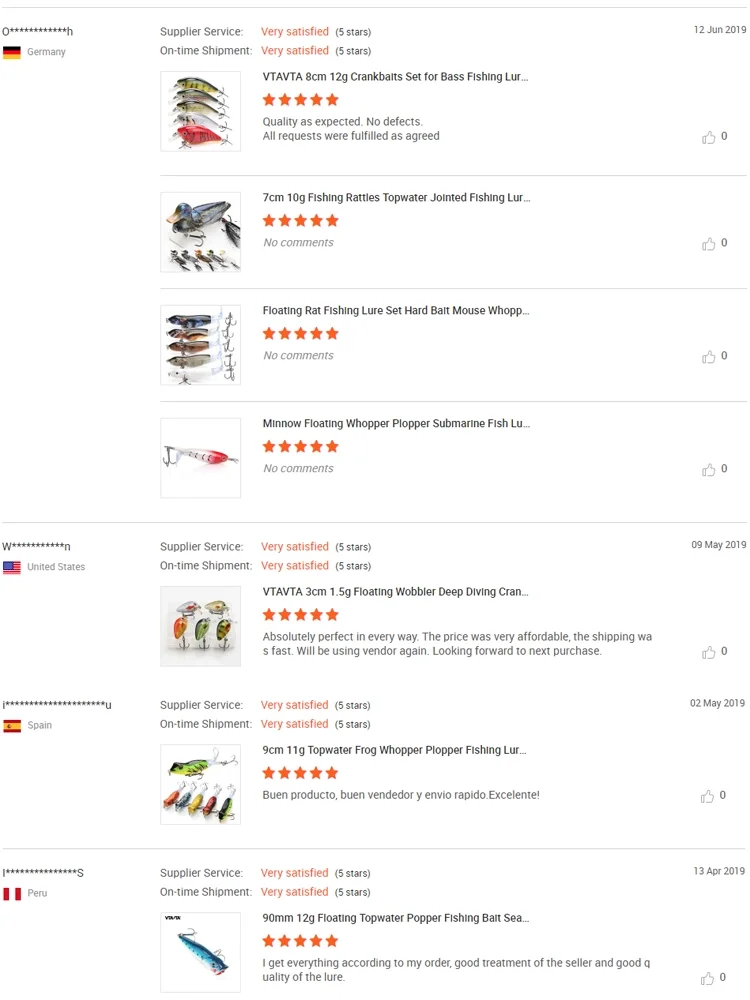The image shows a detailed webpage listing various fishing lures, each accompanied by user ratings and reviews. On the left side, partially obscured usernames are displayed alongside their country of origin and corresponding flags. For example, the first user is from Germany, indicated by a German flag, and has given a "very satisfied" rating with five stars for both the product quality and on-time shipment. 

Displayed prominently is an array of lures from the brand VTVTAVTA, specifically designed for bass fishing. The lures are described as meeting quality expectations with no defects, fulfilling all requested criteria. Each lure in this set has received a consistent five-star rating.

Following this, there is a transition to a review from a user in the United States, who also rates the lures with unanimous five stars, commenting that they are "absolutely perfect in every way." The pattern continues with another user from Peru providing excellent feedback, depicting a list showcasing highly-rated fishing lures that are favored by users from diverse locations.